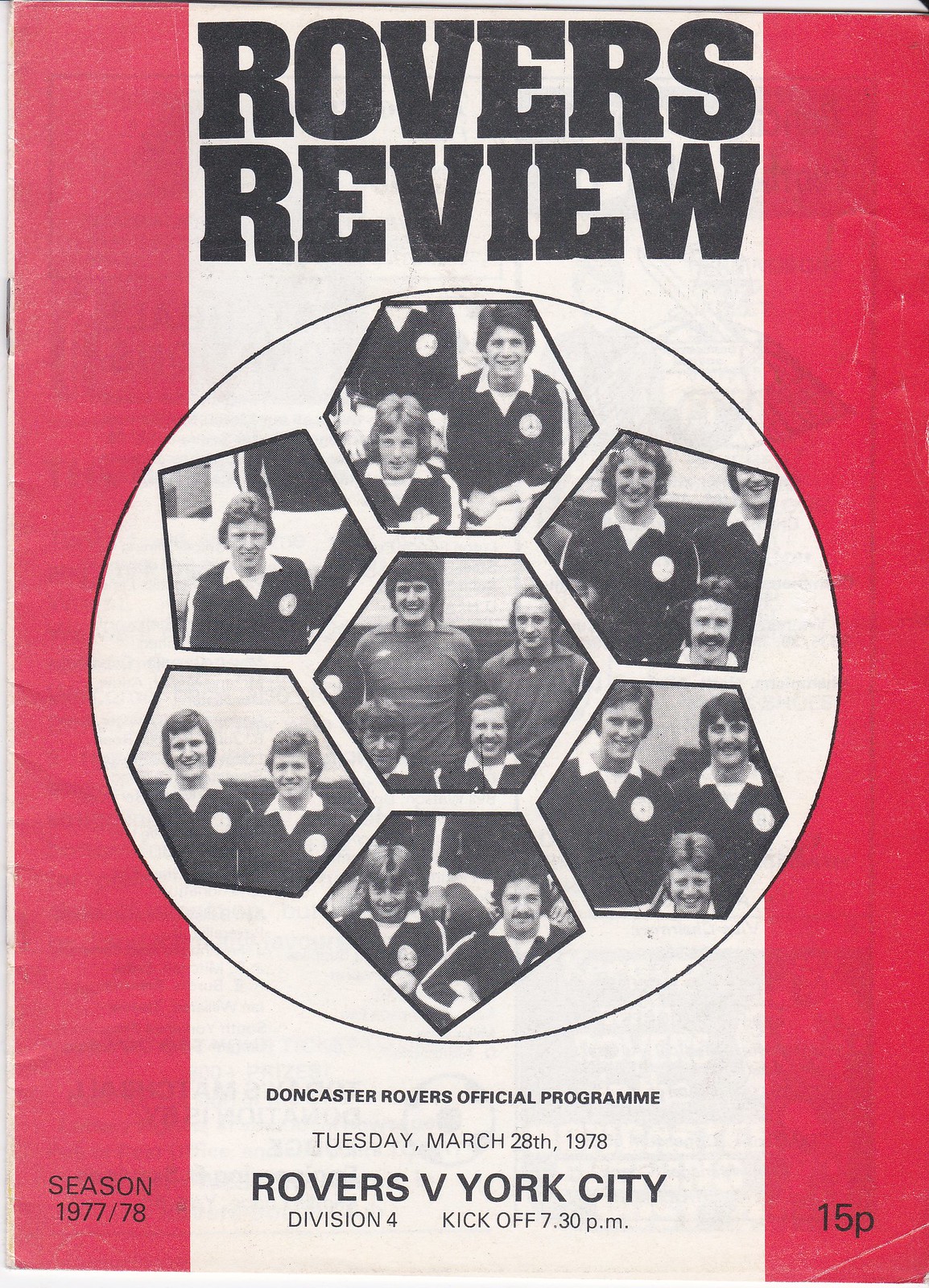The image depicts the front cover of a magazine or newspaper titled "Robur's Review" in large, black, bold capital letters at the very top. The layout is bordered by thin, vertical red bars on both the left and right edges of the page. In the bottom left corner of the left red bar, it reads "Season 1977/78," while the bottom right corner displays "15P." Dominating the center of the cover is a circular collage of black-and-white photos, likely featuring sports players, enclosed in various shapes. Below the collage, the text in black reads "Doncaster Rovers Official Program, Tuesday, March 28th, 1978." Further down, it announces "Rovers v. York City, Division 4, Kickoff 7.30 PM." The vintage style of the cover, characterized by its date and photographic style, indicates that this is a program for a football match, reflective of the late 1970s era.